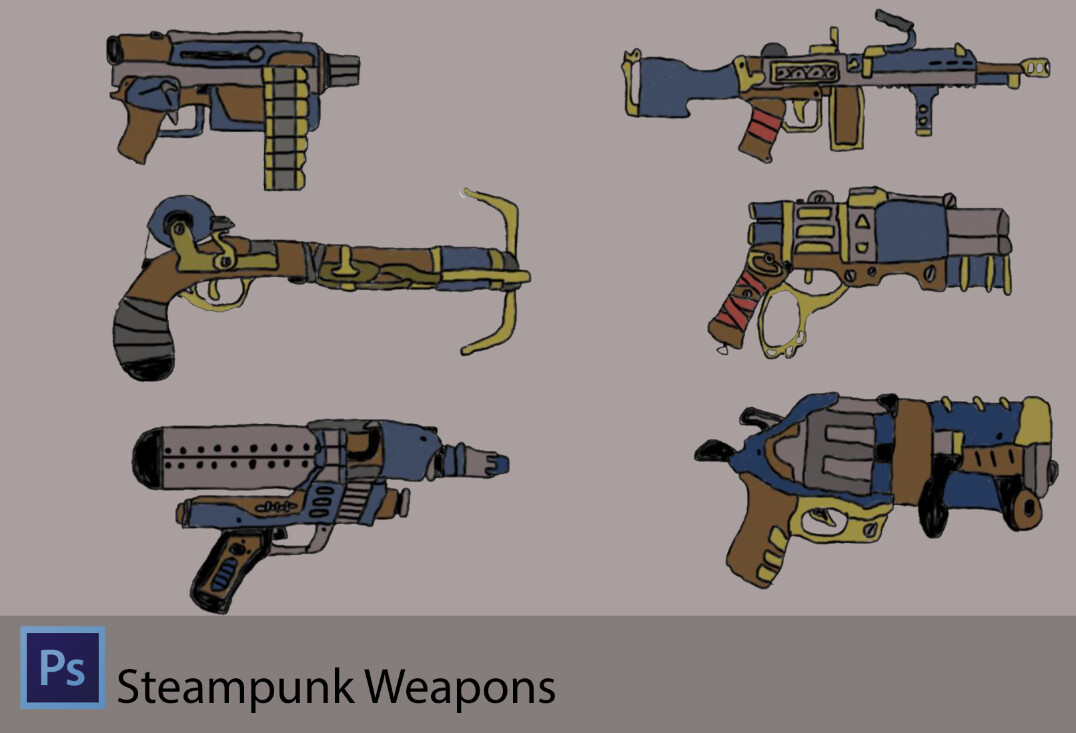The image is a hand-drawn diagram of six distinct, digitally-rendered steampunk-style guns set against a gray background. Each weapon features a palette of gray, black, blue, and brown, with some integrating additional details in yellow or red. Notably, at the bottom of the image, there's a darker gray rectangle housing the black text "STEAMPUNK WEAPONS" alongside a light and dark blue square icon displaying a capital 'P' and a small 's', recognizable as the Photoshop logo.

The top left weapon, similar in length to an Uzi, displays a distinctive pistol shape with colors of brown, blue, and gray, and includes a bullet belt extending downward near the muzzle. Directly below it is a harpoon gun, adorned in blue, gold, brown, and gray, featuring a gold-colored harpoon tip. Next is a drill-shaped gun characterized by a consistent color scheme of gray, black, blue, and brown.

On the right side, there are three more guns. The uppermost resembles a modified AK with a shortened barrel and dual hand grips; the upper grip is gray while the lower one is blue, with an additional brown grip near the muzzle. Below this is a pistol-like weapon in brown, blue, gold, and gray. The bottom-most gun is another pistol variant, predominantly gray with brown and blue accents, and a gold-colored handle. These fantasy weapons exhibit intricate designs and imaginative features, making them resemble elaborate toys rather than real firearms.